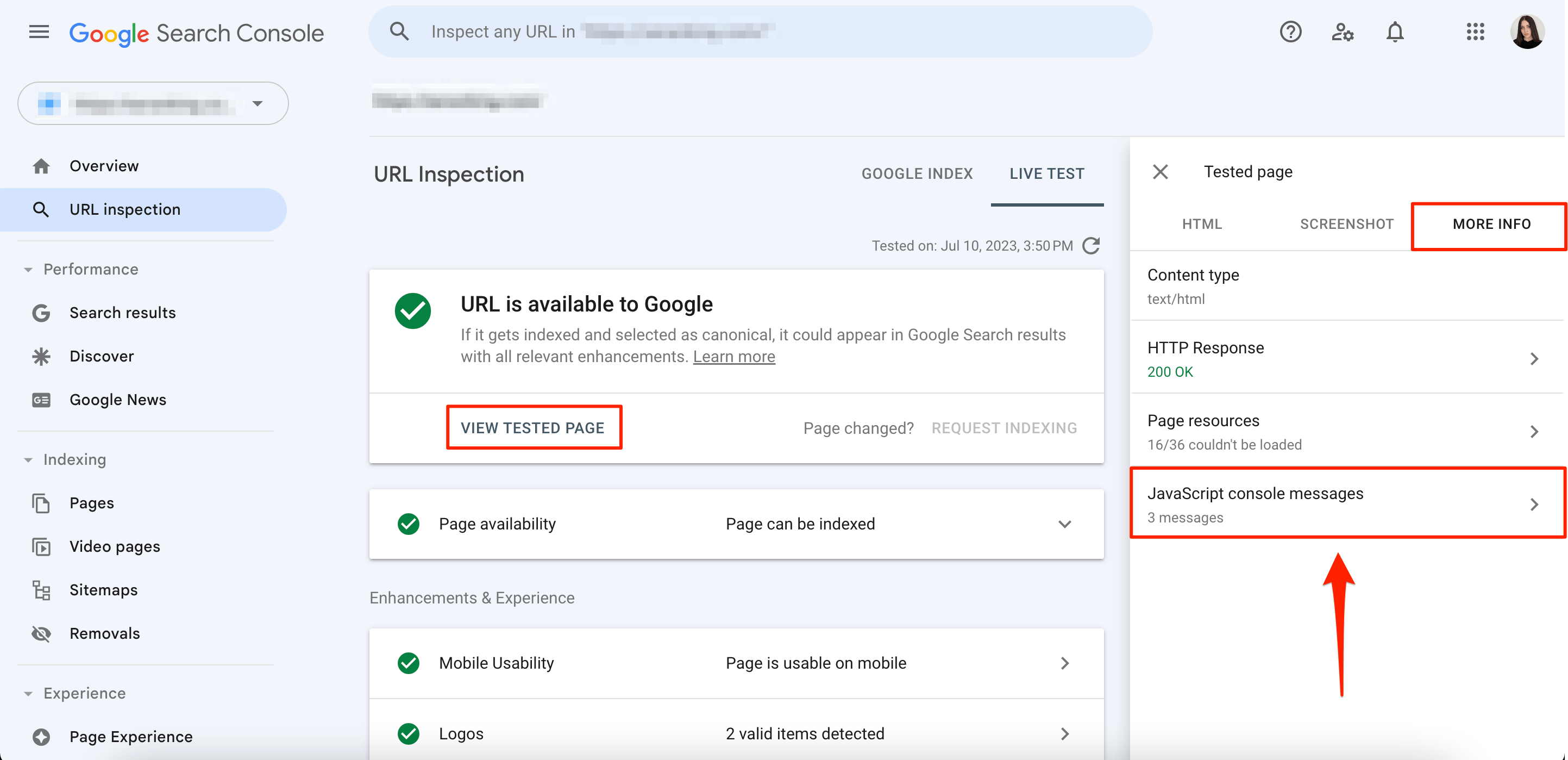Screenshot of Google Search Console: Detailed View and URL Inspection

The image is a screenshot of the Google Search Console interface. At the top-left corner, you can see the Google Search Console logo, followed by a hamburger menu icon. To the right of the logo, there are a series of icons: a bell icon, a grid icon, and a user profile photo situated at the far-right. A light blue search bar is located in the upper section, designated to input and inspect any URL.

The main content area reveals that portions have been pixelated out, including some results and headlines. On the left side, a vertical navigation bar is present, also partially pixelated. At the top of this bar, a home icon is visible, labeled 'Overview'. Below it, the 'URL Inspection' option is selected and highlighted in blue, indicating it's the current active window. Other menu options listed below include 'Performance', 'Search Results', 'Discover', 'Google News', 'Indexing', 'Page', 'Video Pages', 'Sitemaps', and 'Removals'.

The right side of the screen shows the 'URL Inspection' results, organized into several panels. These panels predominantly feature green circles with check marks, affirming that the URL is available to Google. Additional messages indicate that if the URL is indexed and selected as canonical, it could appear in Google search results with all relevant enhancements. A red outline emphasizes the 'View Tested Page' option, suggesting further actions.

To the far right, a panel provides detailed information under the 'Tested Page' heading. This includes an HTML screenshot and a 'More Info' link, which has been highlighted. Further details below this section comprise 'Content Type', 'HTTP Response', 'Page Resources', 'JavaScript Console Messages' (indicated as three messages and outlined in red), and an upward-pointing arrow graphic emanates from beneath this area, drawing attention.

This comprehensive capture of the Google Search Console's 'URL Inspection' tool offers a vivid depiction of its various functionalities and user interface elements.